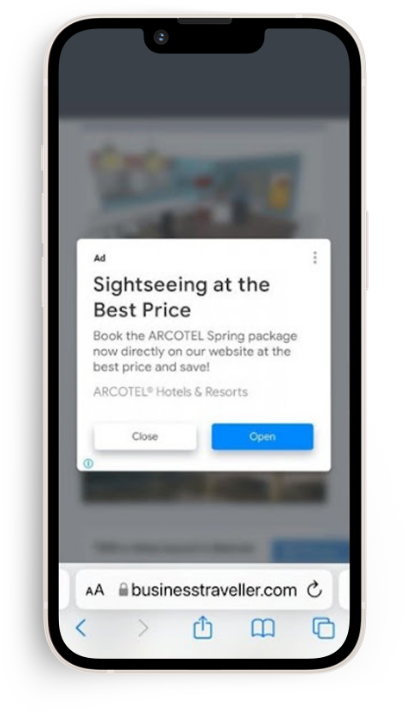**Detailed Caption:**

On a white background, there is a box labeled "Flag as Inappropriate" positioned in the upper left corner. The image prominently features a partially blurry cell phone screen displaying an online advertisement. The ad promotes a deal for "Sightseeing at the Best Price," urging viewers to "Book the Arcatel Spring Package now directly on our website at the best price and save." The ad is for Arcatel Hotels and Resorts. Two buttons are visible: a white button labeled "Close" and a blue button labeled "Open," with the "Open" button appearing to have been activated.

At the bottom of the cell phone screen, the search bar contains icons indicative of text formatting: a small 'A' and a large 'A' for adjusting text size. A lock icon, symbolizing privacy and security, is also present, and the URL "businesstraveler.com" has been selected. Furthermore, there are several function icons including a blue-green arrow, a share icon, a read mode icon, and another unidentified icon, all located at the bottom edge of the screen.

In the blurred background, there is a vibrant, colorful image that seems to be part of a marketing campaign. This visual context adds a splash of color behind the primary elements of the cell phone screen.